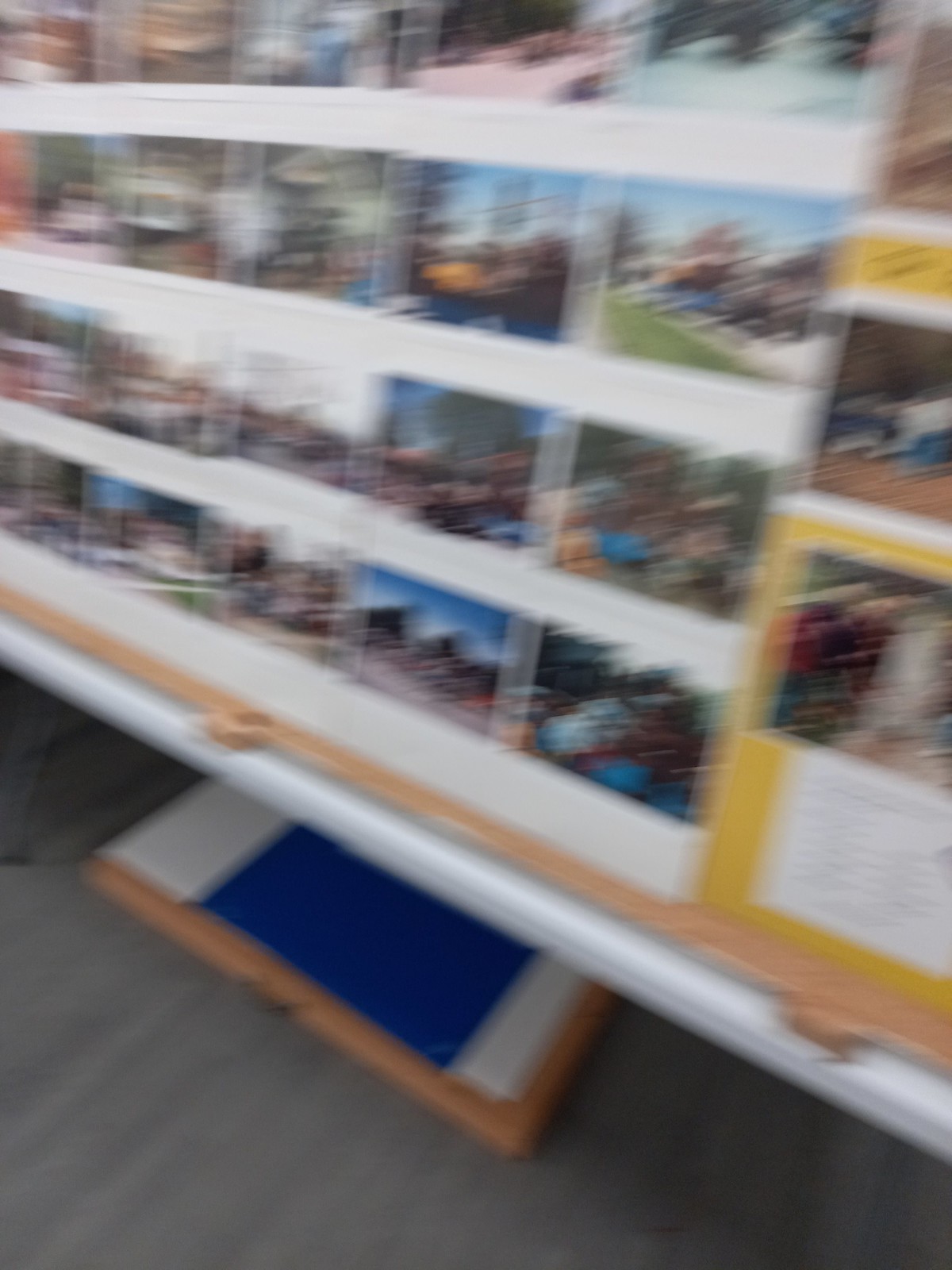The image depicts a somewhat blurry scene of an intricate wall display, reminiscent of a large diorama. The white wall on the left side is covered with various pictures, creating a lively collage. To the right, there's another section filled with more photographs, set against a yellow background. The images predominantly feature outdoor scenes, showcasing blue skies, trees, grass, and groups of people gathered together. Beneath the display, there is a ground-level platform with distinct sections: a brownish outer ring, a blue center, and white sides. The ground itself is a grayish hue, complementing the diverse and colorful spectacle above.